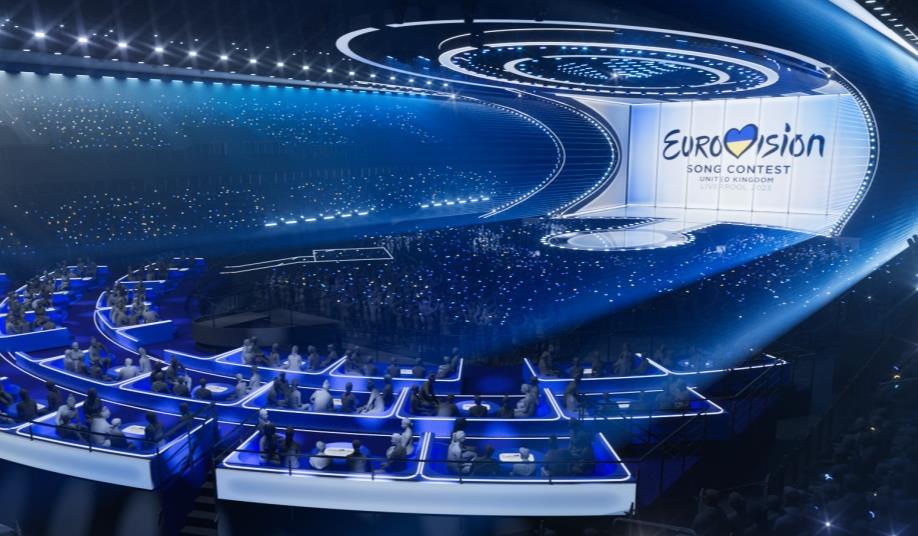The image is a full-color photograph taken indoors under artificial light, capturing a still from the Eurovision Song Contest television program. The photograph is horizontally rectangular and appears to be taken from an elevated position at the back of a large, covered arena filled with blue and white lights. 

In the center of the image is a brightly lit stage, featuring a prominent circular extension designed to facilitate interaction with the audience. The rear of the stage showcases a large sign with the Eurovision Song Contest logo, where the 'V' is creatively shaped like a heart filled with blue and yellow colors. Below the logo, the words "Song Contest United Kingdom" are displayed.

The audience area surrounding the stage is filled with people, many of whom are standing in the general stands, illuminated by a mixture of white and blue lighting that adds a star-like ambiance to the setting. Among the audience, there are several white boxes or compartments; each contains small groups of two to four people seated around tables. These seated sections might be reserved for special guests or judges, adding a sense of organized seating within the larger, bustling crowd.

Overall, the photograph captures the vibrant and bustling atmosphere of the Eurovision Song Contest, highlighting both the grandeur of the stage and the engaged audience.